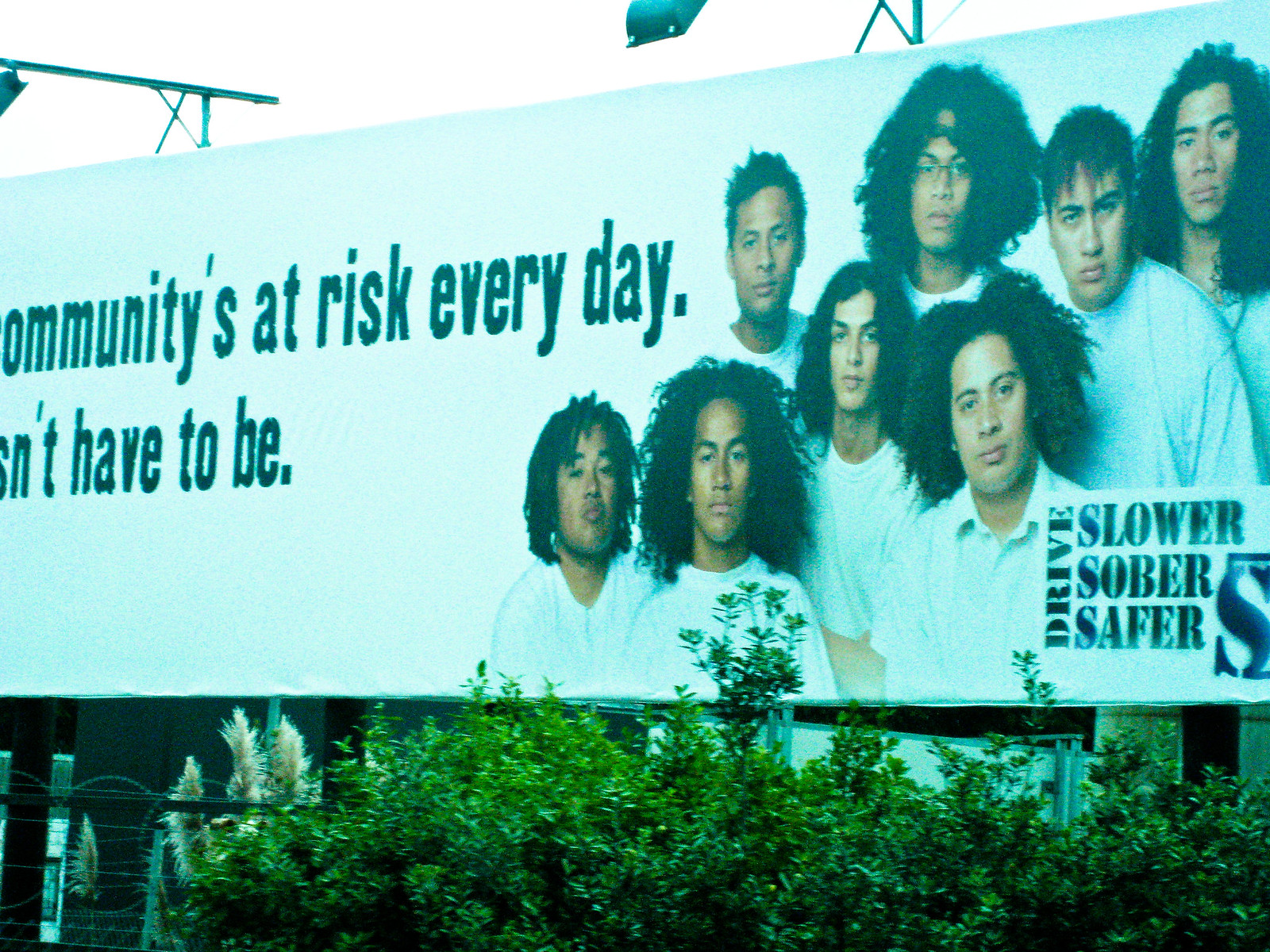A massive, mounted billboard with a long rectangular shape, featuring a white border and background. On the left-hand side, prominently displayed in dark green text, is a slogan that reads: "Communities at risk every day... doesn't have to be." However, the beginning of the slogan is not visible in the image. 

The right-hand side of the billboard showcases a group of young black men, all dressed in white t-shirts. Most of them have loose afros or shoulder-length hair, with a couple sporting shorter hairstyles. All the individuals appear to be quite handsome and are standing together, creating a sense of unity.

In the bottom right-hand corner of the billboard, there's a distinctive logo consisting of the word "DRIVE" written in a vertical orientation with the letters stacked upward. Alongside this, another slogan reads, "sober, slower, safer," emphasizing the campaign's message. The design is anchored by a large, prominent letter "S," reinforcing the theme of safety and caution.